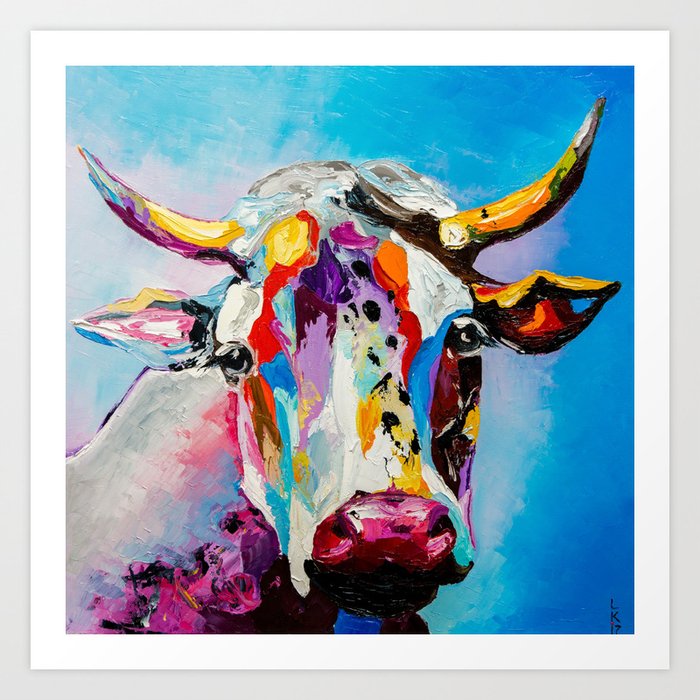Displayed against an off-white colored wall, this photograph features an elaborate painting on a white canvas. The canvas itself is surrounded by a light gray border, followed by a white inner border. At the center of this setting is a strikingly colorful and abstract portrait of a cow's face, set against a blue backdrop. The cow's face and body are a vivid blend of multiple colors: its nose is predominantly pink, while its surrounding area transitions into whites and yellows. The area around the eyes features blues and reds, adding to the intricate pattern. 

The cow's horns, prominently painted in yellows near the base, transition to a mix of purple, white, and green towards the tips. The right horn, in particular, has noticeable black markings extending from the head towards the ear, while the left horn is predominantly purple. The ears are equally colorful, with the right ear displaying a yellow outline on top, black at the bottom, and red and blue within. In contrast, the left ear showcases a yellow and blue outline with a black inner outline near the head, and a purple and white interior.

Detailed further, the forehead exhibits a mix of purple, yellow, and orange spots. Black dots embellish the middle of the cow's face, adding depth and contrast. The right eye is positioned slightly farther left of center compared to the right eye. The cow’s mouth and surrounding areas display shades of purple, with black features extending below, suggesting either a part of the nose or a body outline. 

The cow's neck and upper body are primarily white, transitioning to blue and brown shades. Notably, smaller details such as the black initials "LK17" appear vertically in the bottom right corner of the painting. Overall, the piece vividly captures an abstract and vibrant representation of a cow's face amidst a blue background.